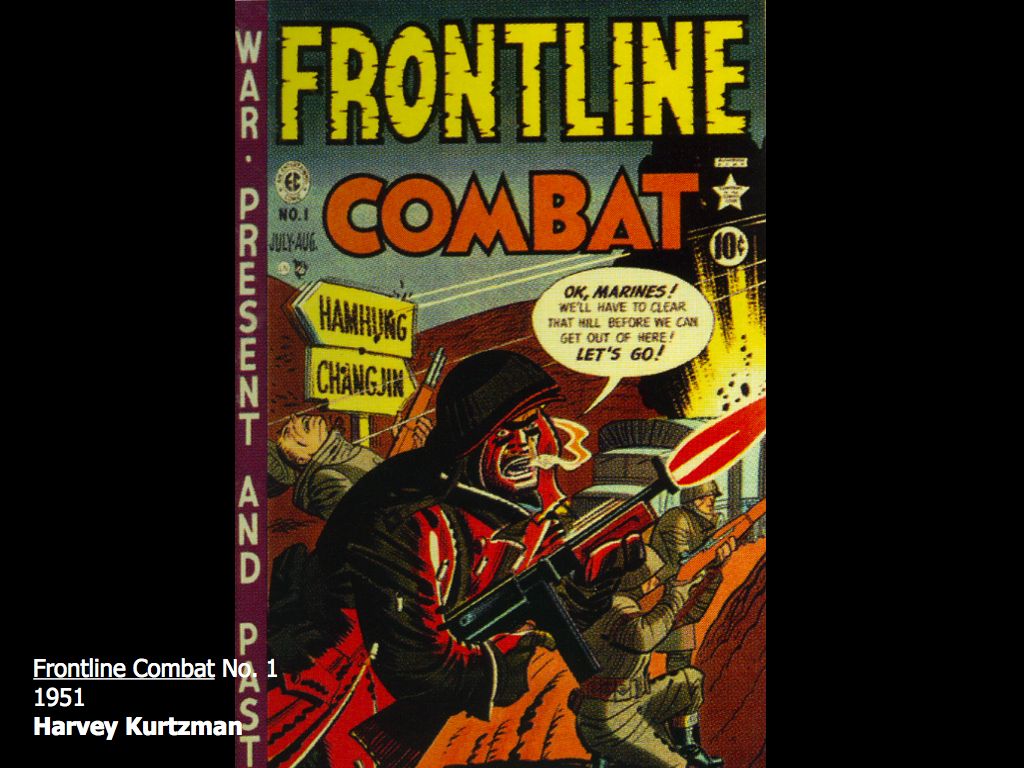The image depicts the cover of a comic book titled "Frontline Combat No. 1, 1951, Harvey Kurtzman," characterized by a dramatic portrayal of wartime action. The cover features a central figure, a man dressed in all black, firing an automatic rifle with rapid bursts of gunfire. This soldier, who appears to be giving commands, is captured in the midst of action with a word bubble stating, "Okay, Marines, we'll have to clear that hill before we can get out of here. Let's go."

The scene extends to the background where additional soldiers are engaged in intense combat. On the bottom right, two more soldiers are depicted, with one near a military vehicle that is exploding. On the left side, a soldier is seen recoiling, likely after getting shot. The overall imagery is border-framed, with black edges on both sides and a purple spine border. The text "War, Present, and Past" prominently runs down the spine, and the title "Frontline Combat" is split with "Frontline" in yellow font and "Combat" in orange. Some text is written in a different language, and there is a star graphic on the left side of the cover.